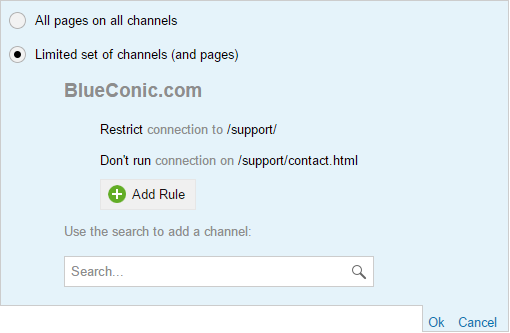The image depicts a segmented web page with a gray border and a light blue background. At the top left, there are two radio button options: "All pages on all channels" and the selected "Limited set of channels (and pages)". Below, the text "blueconic.com" is visible, followed by "connect/connect to/support/". On the next line, it reads "Don't run connection on/support/contact.html". A green circular button with a white plus sign inside appears below this text, followed by the option to "Add rule" to the right of the button. Underneath, the text instructs users to "Use the search to add a channel", accompanied by a search box and a magnifying glass icon on the right. Finally, in the lower right corner, there are blue "OK" and "Cancel" buttons. The user is unfamiliar with the website blueconic.com, speculating it might be related to setting up a YouTube channel, though this is uncertain.